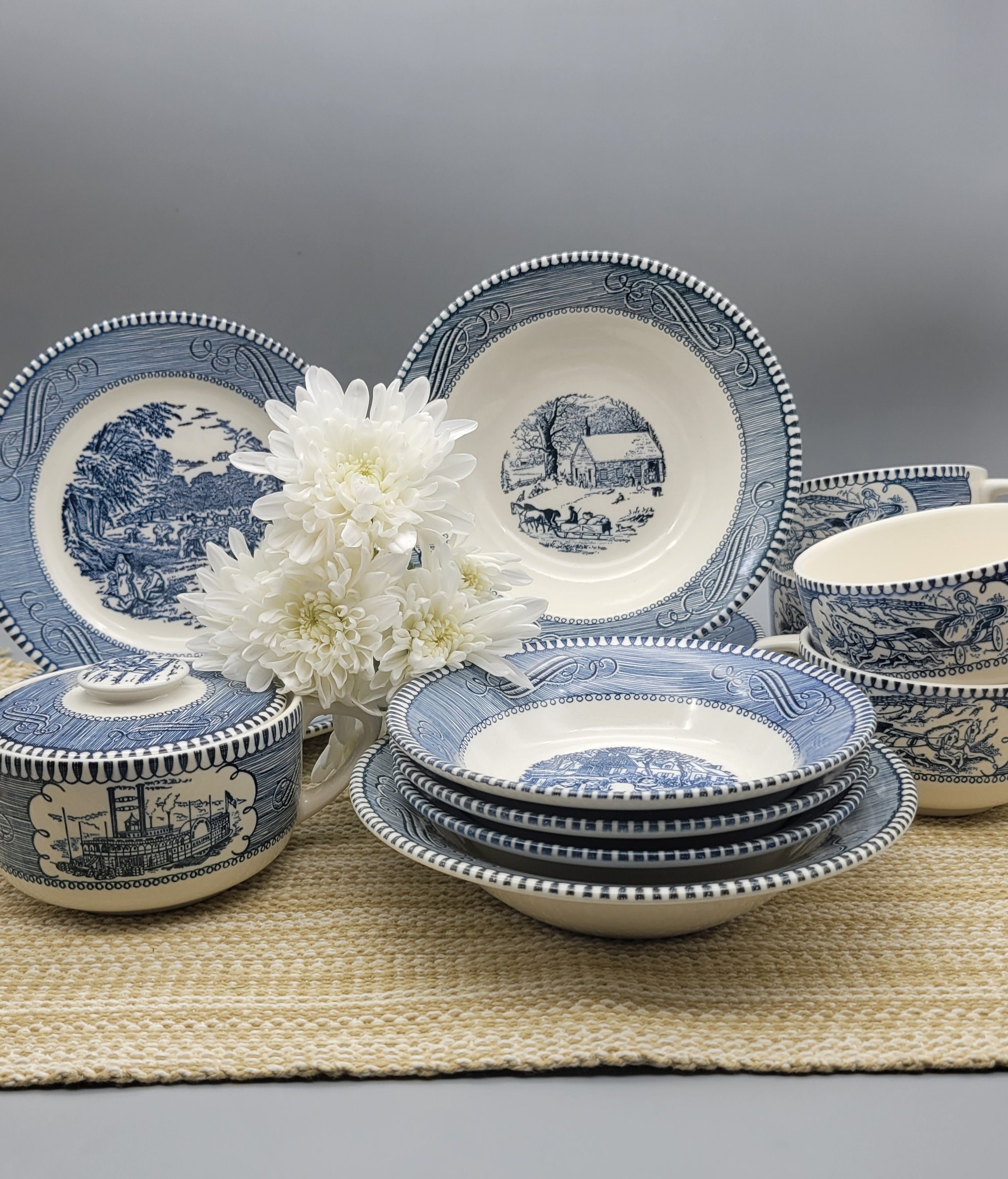The image depicts a meticulously arranged set of fine china reminiscent of Williamsburg blue pottery from the 1980s. Central to this display are intricate illustrations in blue, featuring scenes such as colonial buildings, landscapes with trees, and ships surrounded by a clear white space. These designs are encircled by distinctive blue and white patterned borders. The set includes various pieces: two plates displayed upright at the back, bowls stacked atop each other at the front, and tea cups or coffee cups, some covered, arranged to the right. Additionally, a small pot and possibly a sugar bowl or creamer sit to the left. The entire arrangement rests on a beige rattan table runner that spans a gray tabletop, accentuating the elegant blue and white china pieces. The setting is further adorned with white flowers, adding a delicate touch to the composition.